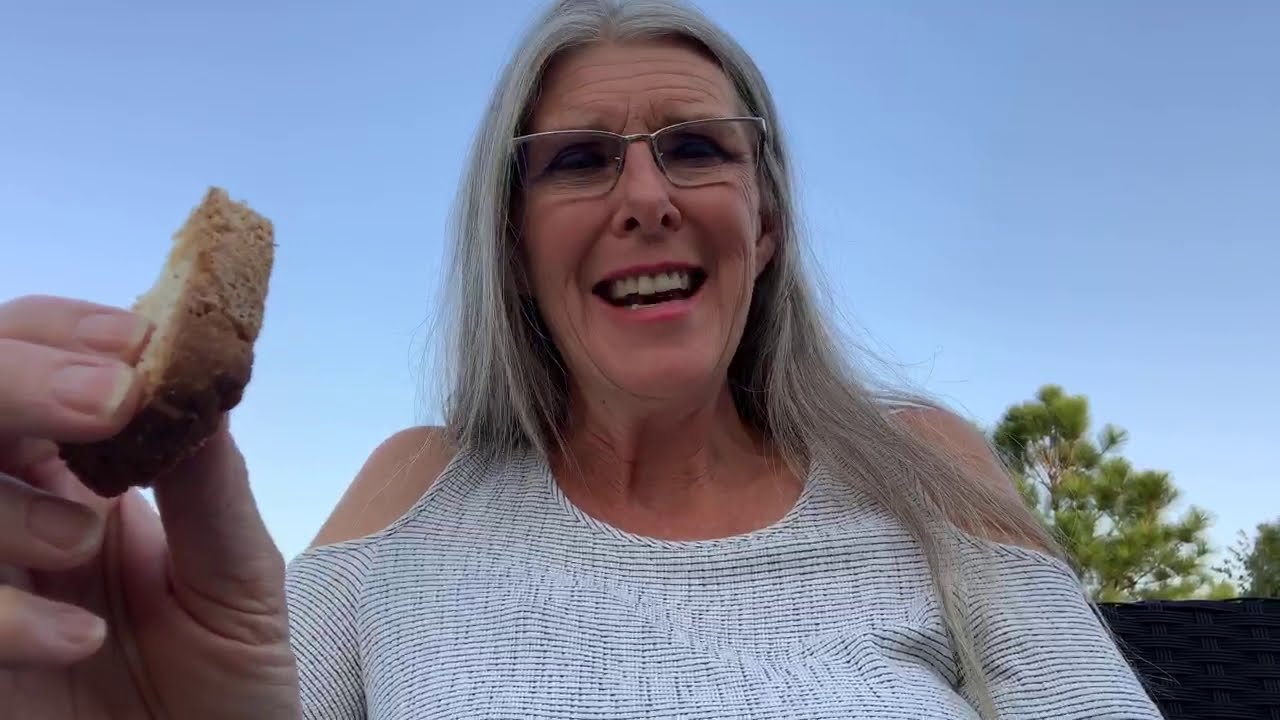The image depicts an older woman, likely in her 60s, who appears to be having a joyful moment outdoors. She has long gray hair and is wearing glasses along with a white and gray striped top. The woman, who has a piece of bread with a brown crust in her right hand, is either smiling or laughing with her mouth open, revealing her teeth. Her peach-toned skin and well-groomed nails are also visible. Seated comfortably on a black outdoor chair, she is surrounded by a serene setting with a blue daytime sky and distant green pine trees. The overall atmosphere suggests a pleasant, relaxed spring or summer day, with the woman radiating happiness and possibly enjoying a meal, perhaps brunch, in an outdoor setting. The vibrant colors of the scene include the blue sky, the green trees, and the earthy browns of the bread, adding to the image's cheerful and tranquil mood.